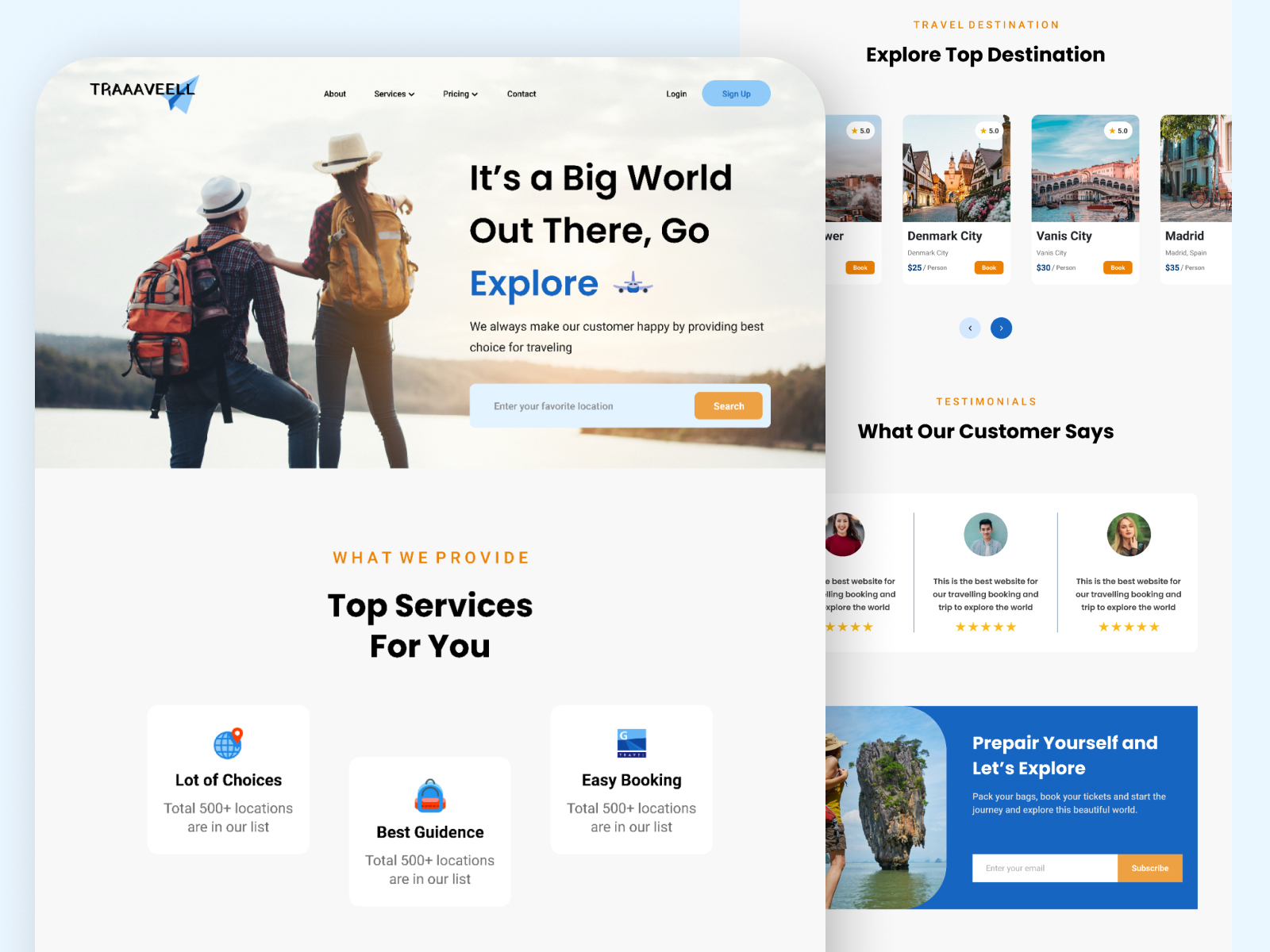Screenshot of Travel Web Page:

In the upper left-hand corner, the word "Travelllee" is prominently displayed, creatively elongated with three A's, two E's, and two L's. A blue triangular shape partially overlays the E and L's, pointing towards the upper right. The top menu includes navigation options such as About, Services, Pricing, and Contact, along with buttons for Log In and Sign Up.

The central focus of the screenshot is a captivating photo of a man and a woman standing side by side, gazing out over a serene body of water with rolling hills beyond. Viewed from behind, the man on the left sports a white hat, a plaid shirt, blue jeans, and an orange backpack. The woman, also viewed from behind, wears a beige straw hat and has long brown hair. She carries an orange backpack similar to the man's, paired with a plaid shirt and dark-colored jeans. 

To the right of the photo, the text reads, "It's a big world out there. Go explore," accompanied by a small plane logo. Below this inspiring tagline, additional promotional text promises customer satisfaction by offering the best travel choices and encourages users to enter their favorite locations to explore what the site provides. Key service highlights include "Top services for you," "500+ locations on our list," "Best guidance," and "Easy booking."

This section of the web page is positioned over another part of the interface, which extends into the right of the screenshot, though details of that portion are obscured.